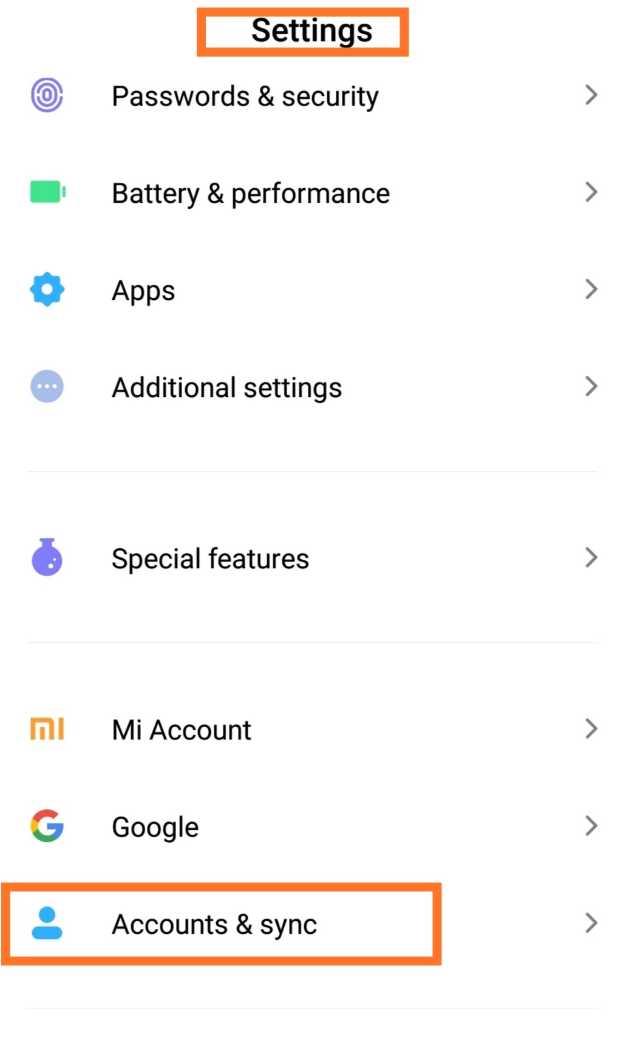The image depicts a settings webpage outlined in an orange box. The webpage is organized into several sections, each with an associated icon and text. 

At the top, highlighted by an orange box, is the title "Settings." Below this, the first section reads "Passwords and Security," marked by a purple icon. This is followed by "Battery and Performance" featuring a green icon. Next in line is "Apps," denoted with a blue icon, and then "Additional Settings" with a light purple icon.

A thin gray line separates these sections from the next category titled "Special Features," which includes a purple icon beside it. Another division marked by a thin gray line introduces the subsequent section labeled "MI Account" with an orange image. Following this is "Google," represented by a multicolored 'G'.

At the bottom, the final section is “Account and Sync,” also highlighted by an orange outline. Within this box is a generic blue icon of a person. The entire background of the settings page is white, serving to emphasize the orange-highlighted sections for "Settings" and "Account and Sync."

Overall, the image provides a clear and organized view of the settings menu, with each section distinctly identified by both text and colorful icons.